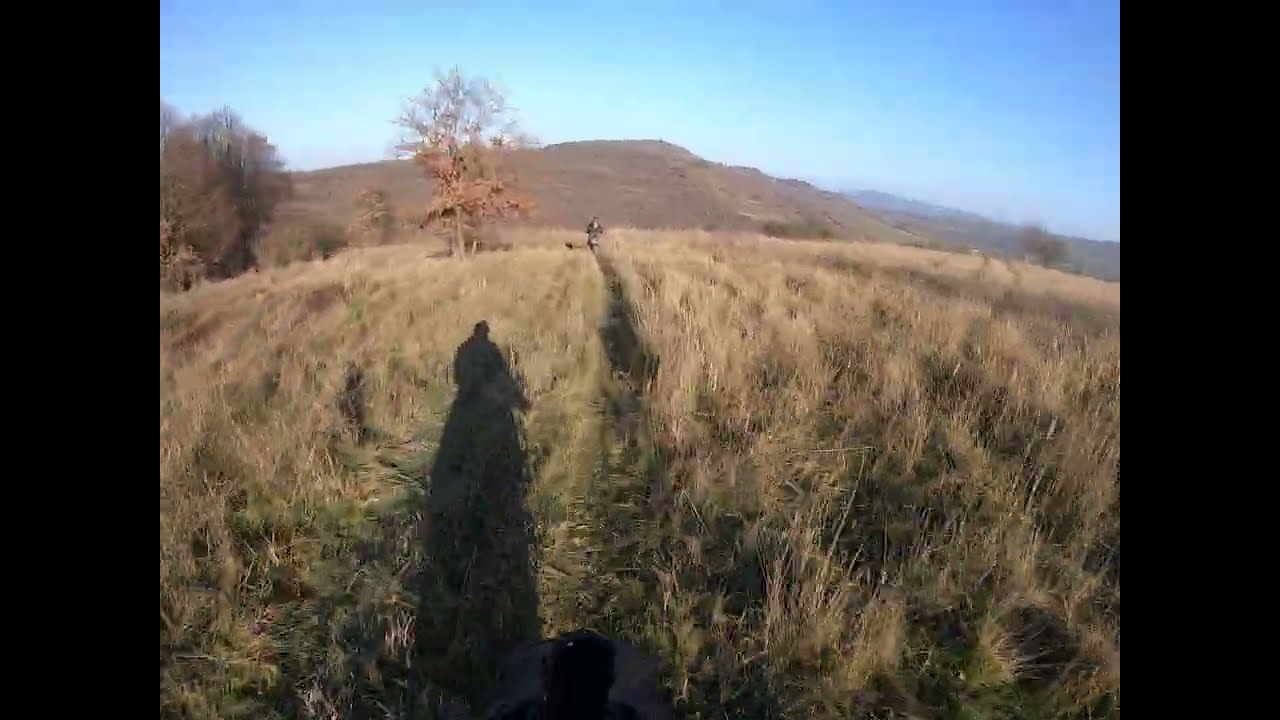In this outdoor daytime image, a vast field with predominantly dead, brown grass about a foot and a half tall stretches out before us. A dirt path cuts through the field, where a person rides a black dirt bike. The field is dotted with multiple trees on the left side; these trees have sparse, dying leaves, indicative of the colder months, with some brown leaves still clinging on. The scene is bathed in sunlight under a clear blue sky, highlighting the natural colors of the landscape - light blue, white, gray, brown, yellow, green, tan, and black. Shadows are cast by the figures and trees in the image. The background features rolling hills and a distant mountain range, adding depth to the sprawling, uncultivated landscape. To the right, another tree stands in the far distance, balancing the composition. The image captures the sprawling, unstructured beauty of the field, focusing more on the overall landscape rather than any particular object, creating a serene and expansive view.